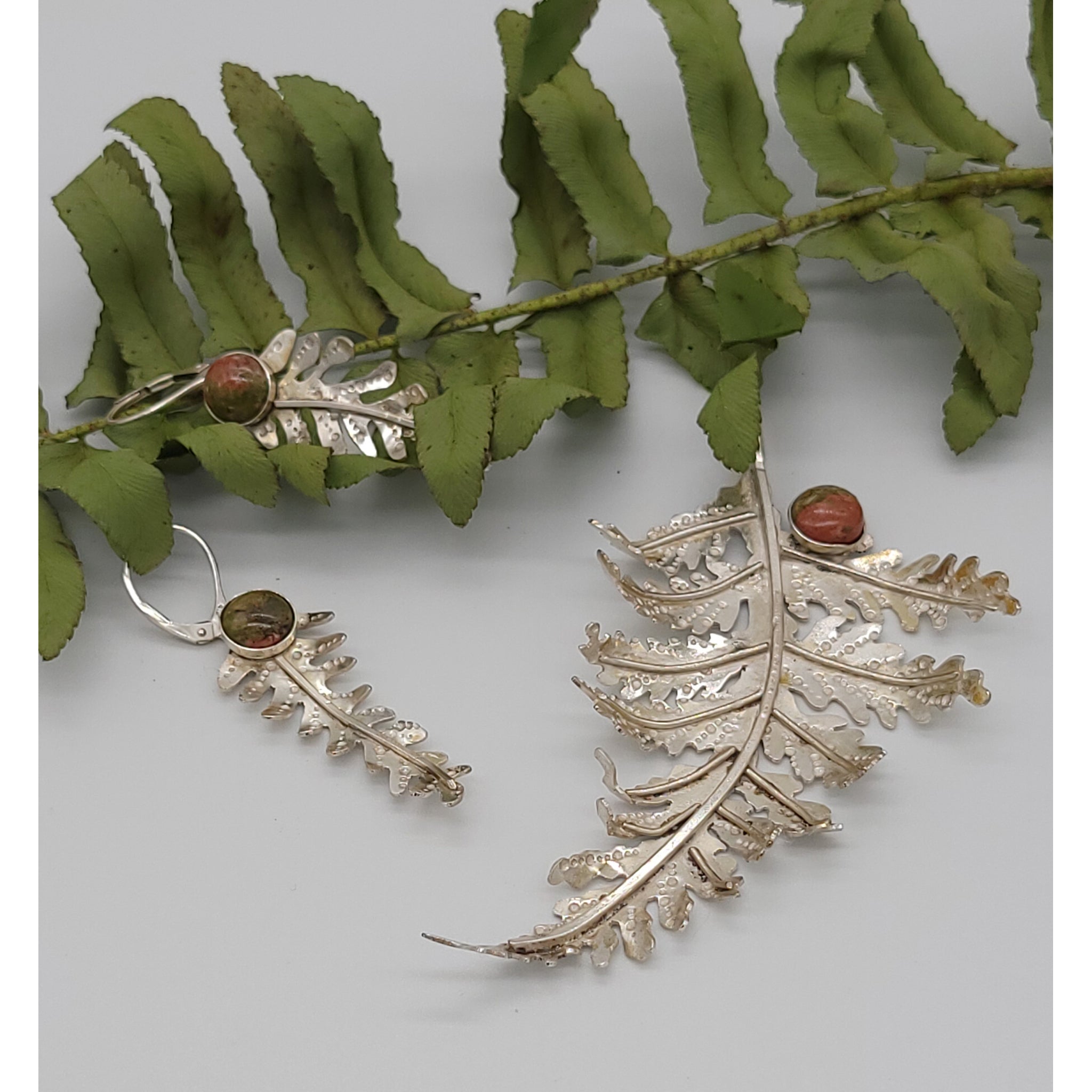In this image, a set of intricately designed jewelry pieces are displayed against a gray background. At the center, a pair of silver-colored earrings shaped like ferns take precedence. Each earring features a delicate, fern-like leaf crafted from shiny, faux silver metal, adorned with a reddish-brown gemstone at the top, where the earring hook begins. The earrings are positioned near a larger matching piece, which resembles a pendant or brooch. This larger fern, made from the same faux silver metal, mirrors the form of the earrings, including a similar reddish-brown gemstone intricately attached to one of its leaves. 

Adding a touch of contrast, artificial green fern leaves extend diagonally across the background, their narrow, elongated fronds made of plastic, accentuating the silver shine and elaborate design of the jewelry.